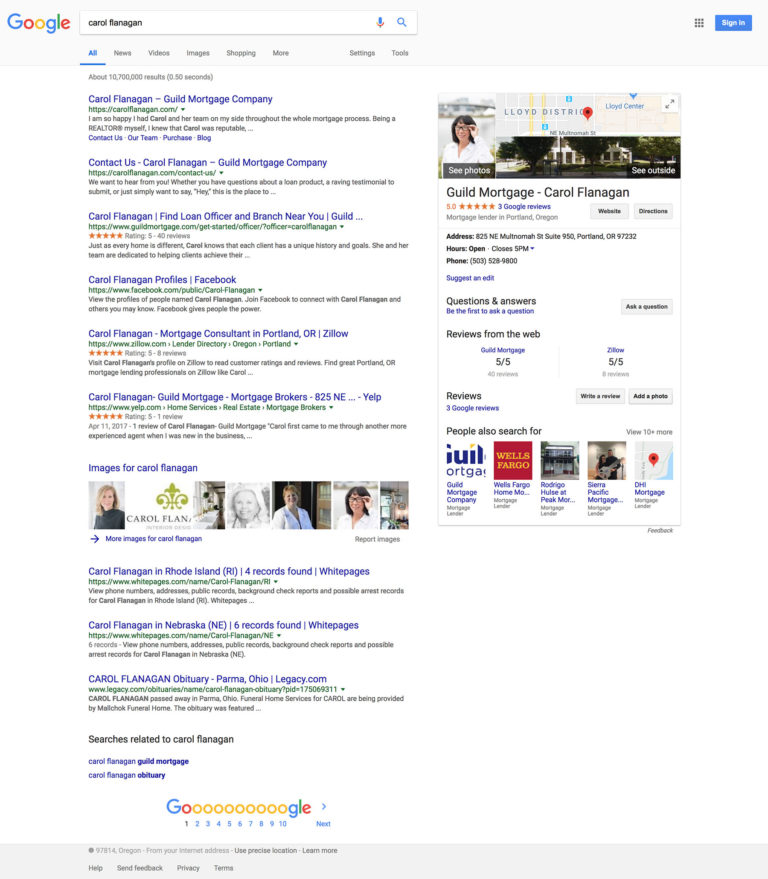This is a detailed screenshot of a Google search results page. The page features a classic gray header with the Google logo prominently displayed on the top left. To the right of the logo is a search bar where the query "Carol Burgess" has been entered. Below the search bar is a navigation menu with categories such as All, Home, Videos, Photos, Shopping, and More. The "All" category is highlighted, indicating that it is currently displaying all available information.

At the center of the page, there are multiple thumbnails of a woman identified as Carol Burgess. To the right of these thumbnails is information related to a Realtor, presumably associated with Carol Burgess. The main section of the page consists of numerous listings displayed vertically, some of which include ratings from Google users. Additionally, on the bottom right of the screenshot, there is a mobile view of the search results page, specifically relating to Carol Burgess, showcasing similar information in a more compact format.